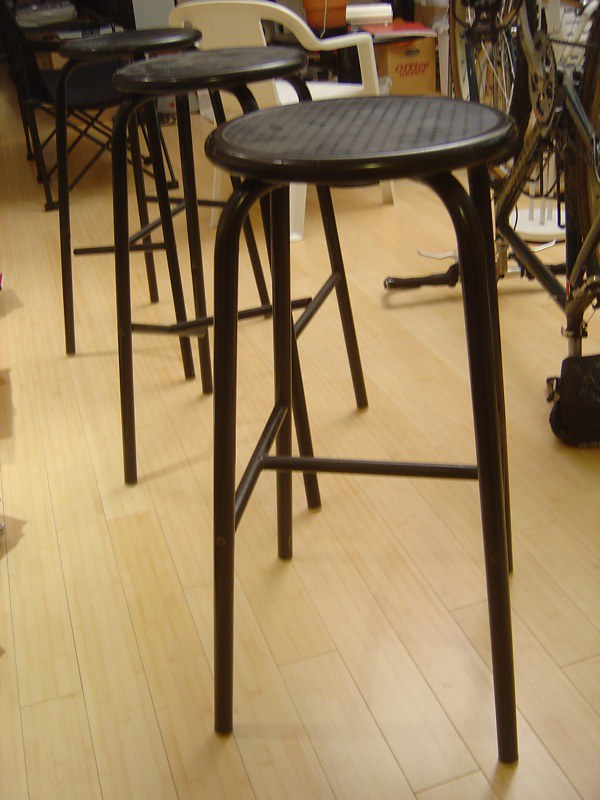The color photograph showcases a room with light brown, blonde-colored wood panel flooring. In the foreground, there are four dark brown or black barstools, each featuring round seats and long, slender legs. These stools are arranged in a line, with one positioned closer to the viewer and the remaining three receding into the background. To the left, a white plastic armchair is visible, and on the right, a cluttered area includes an Office Depot box, an upside-down bicycle, and various other items. The image appears to focus on the barstools, possibly indicating they are the main subject of interest, perhaps for selling or display purposes.